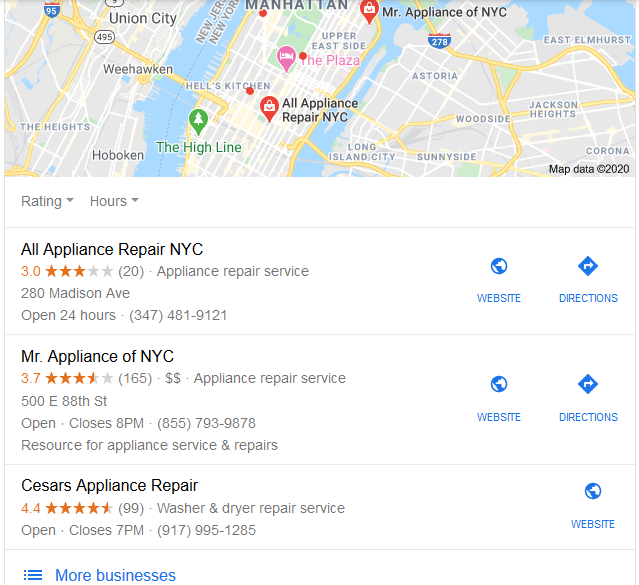This image captures a Google Maps search result in portrait orientation, framed by a border on the top left and right, with the bottom unbordered. The image is slightly taller than it is wide. A rectangular map of New York City spans the top portion of the screen, prominently featuring Manhattan. Landmasses and waterways, including notable locations such as Hoboken, New Jersey, Astoria, and Sunnyside, are clearly visible.

Beneath the map, a series of search results are displayed, each with a black header, a star rating system (with yellow stars against a gray background ranging from 0 to 5), the number of ratings, descriptions, addresses, operating hours, and phone numbers. To the right of each result, blue links offer options to visit the website or get directions. At the very bottom of the search results, a hamburger menu labeled "More businesses" is present.

The search results listed are:
1. **All Appliance Repair:** Rated three stars.
2. **Mr. Appliance of New York City:** Rated 3.7 stars.
3. **Caesars Appliance Repair:** Rated 4.4 stars, making it the highest-rated among the listed options. This establishment specifies that it offers washer and dryer repair services, whereas the other two entries mention general appliance repair services.

The detailed interface provides comprehensive information to help users make an informed choice.